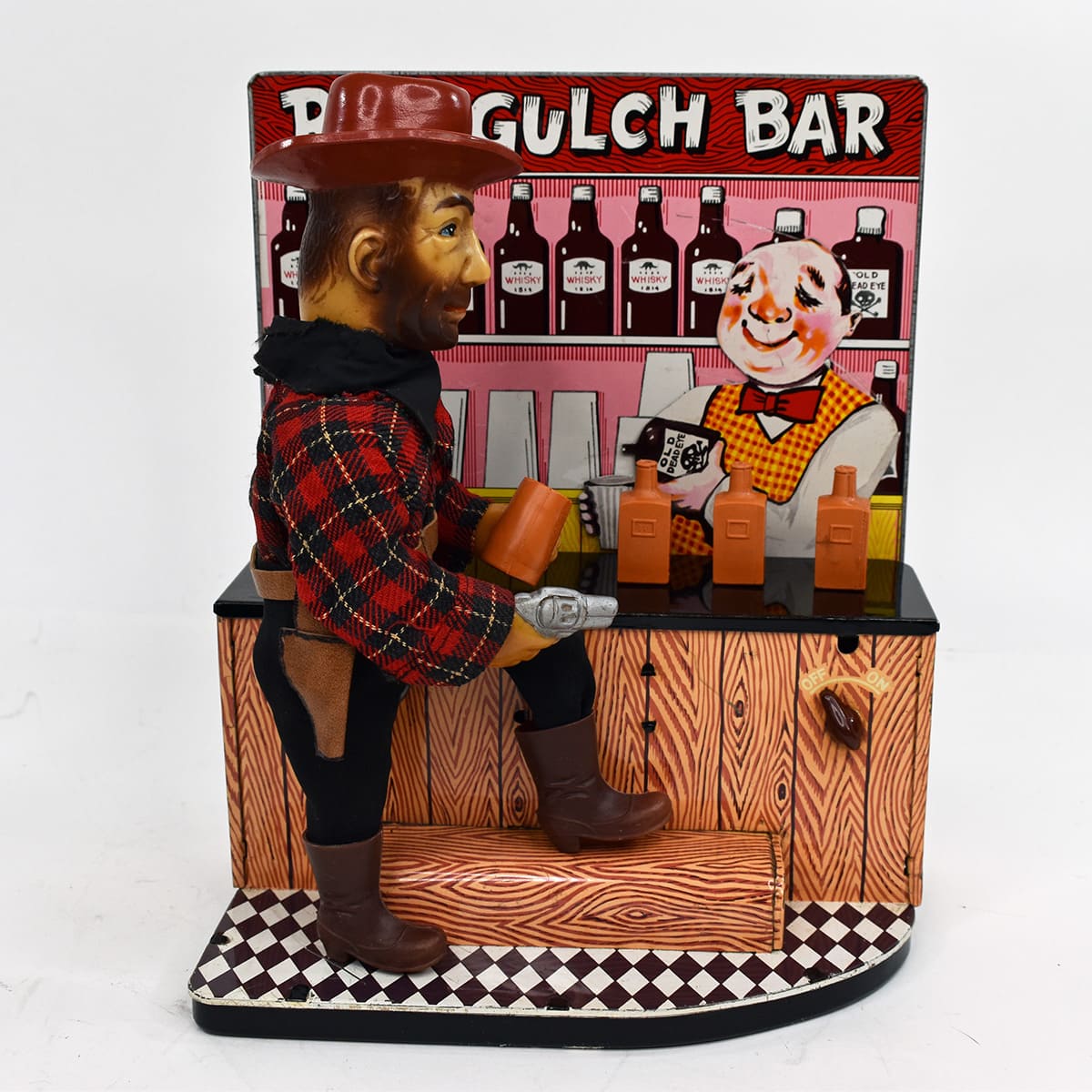The image depicts a vintage mixed media figurine of a cowboy positioned at a bar in the foreground. The cowboy, outfitted in a red plaid long-sleeved shirt, black pants, and brown cowboy boots, sports a full brown beard, short brown hair, and a maroon cowboy hat. He holds a silver pistol in his right hand and a terracotta-colored mug in his left. His left foot rests on a black and white diamond-patterned floor while his right foot is propped on a wooden log at the base of the bar. 

The bar itself features a wood plank front and a black top, complemented by small terracotta figurines of liquor bottles on the right side. Behind the bar, a painted figure of a bartender, dressed in a checkered bib of orange and red, a red bow tie, and a white shirt, is seen pouring a black bottle into a silver cup. This painted backdrop also includes shelves stocked with liquor bottles and cups, with a red border displaying white lettering that spells out "Gulch Bar." An on-off switch is situated to the right side of the bar, currently set to off.